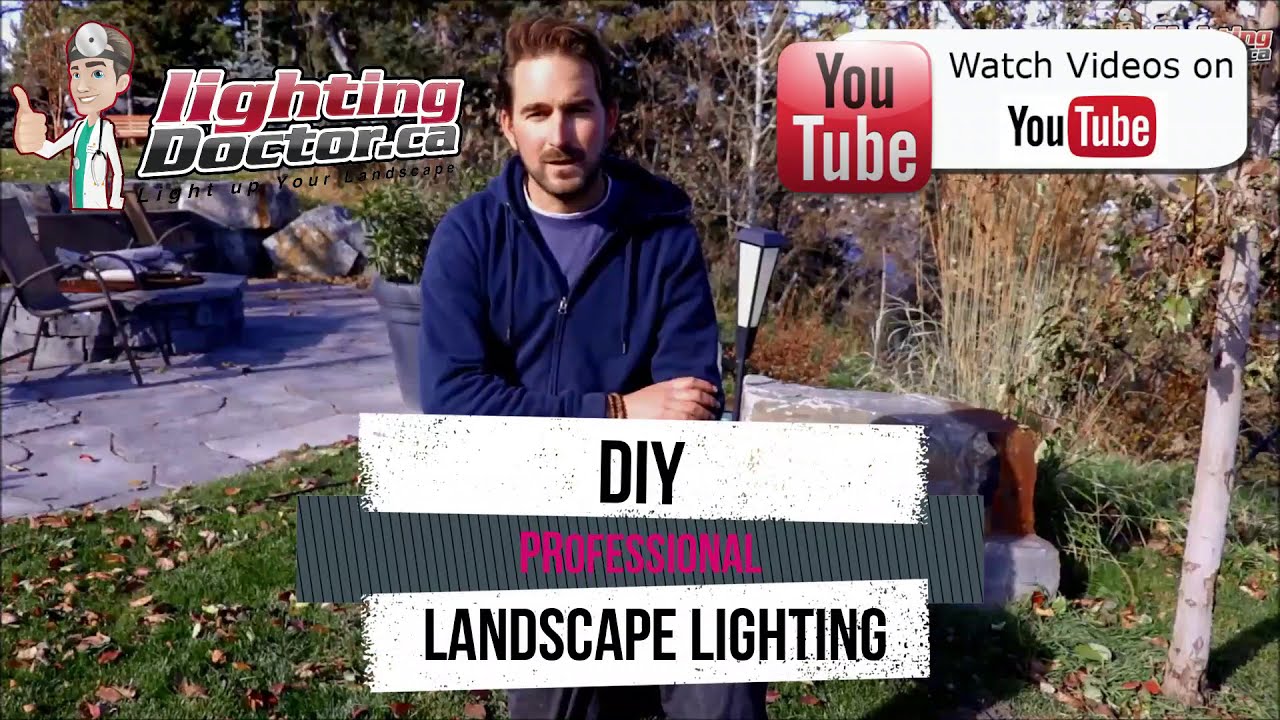The image is a promotional banner for a YouTube channel, featuring a cartoon doctor character in the top left corner, giving a thumbs-up and wearing a doctor's coat and green scrubs, accompanied by the text "lightingdoctor.ca." The banner's slogan, partially obscured, reads, "Lighting up your ...". The top right corner features a YouTube logo with the text, "Watch videos on YouTube." At the bottom center of the banner, "DIY Professional Landscape Lighting" is prominently displayed.

The image captures an outdoor scene with a man in a blue hoodie, standing or sitting on a grassy area adjacent to a gray stone patio equipped with a fire pit and several metal outdoor chairs. The man, who is light-skinned with short brown hair and facial hair, appears to lean on or be near a solar panel set on the ground. The setting is filled with various trees and shrubs in different shades of green, and the ground is littered with brown and red autumn leaves, suggesting a fall season.